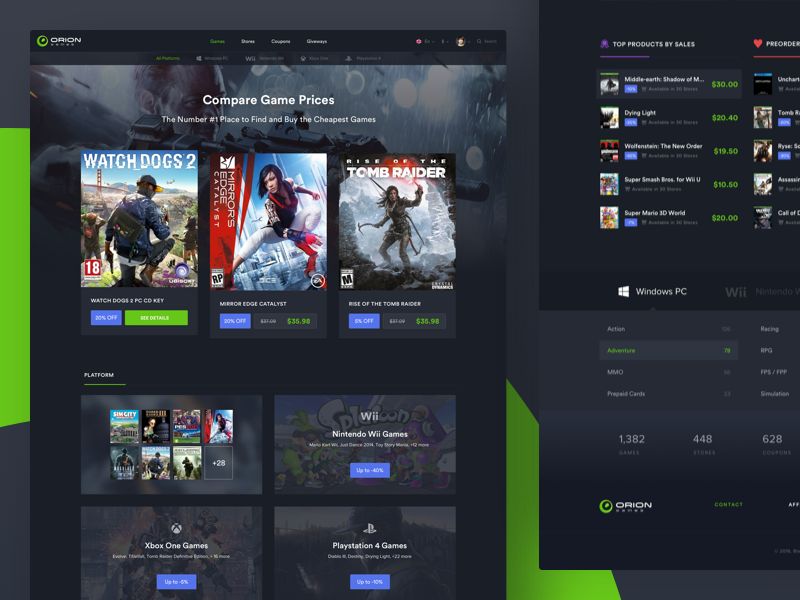The image showcases a display ad featuring two nested screenshots within a rectangular frame. The left section appears to be from a smartphone interface, predominantly characterized by a dark blue background. This section seems to be a webpage designed for purchasing video games. At the top of the screen, beneath an illegible black border, the phrase "compare game prices" is clearly visible in white text. Below this, three games are prominently displayed: Watch Dogs 2, an unidentified game showing a close-up of a man likely engaged in a sword fight, and Tomb Raider, featuring the iconic protagonist set against a tomb-like backdrop. Further down, there are four smaller squares, each containing game titles, although the text is too tiny to decipher.

On the upper right-hand portion of the ad, there is part of another screenshot, possibly from a different page of the same website. This section lists games in a compact format with very small images and text. The games are arranged in two columns; the left column contains five games, while the right column also features five, but the descriptions are partially cropped and difficult to fully discern.